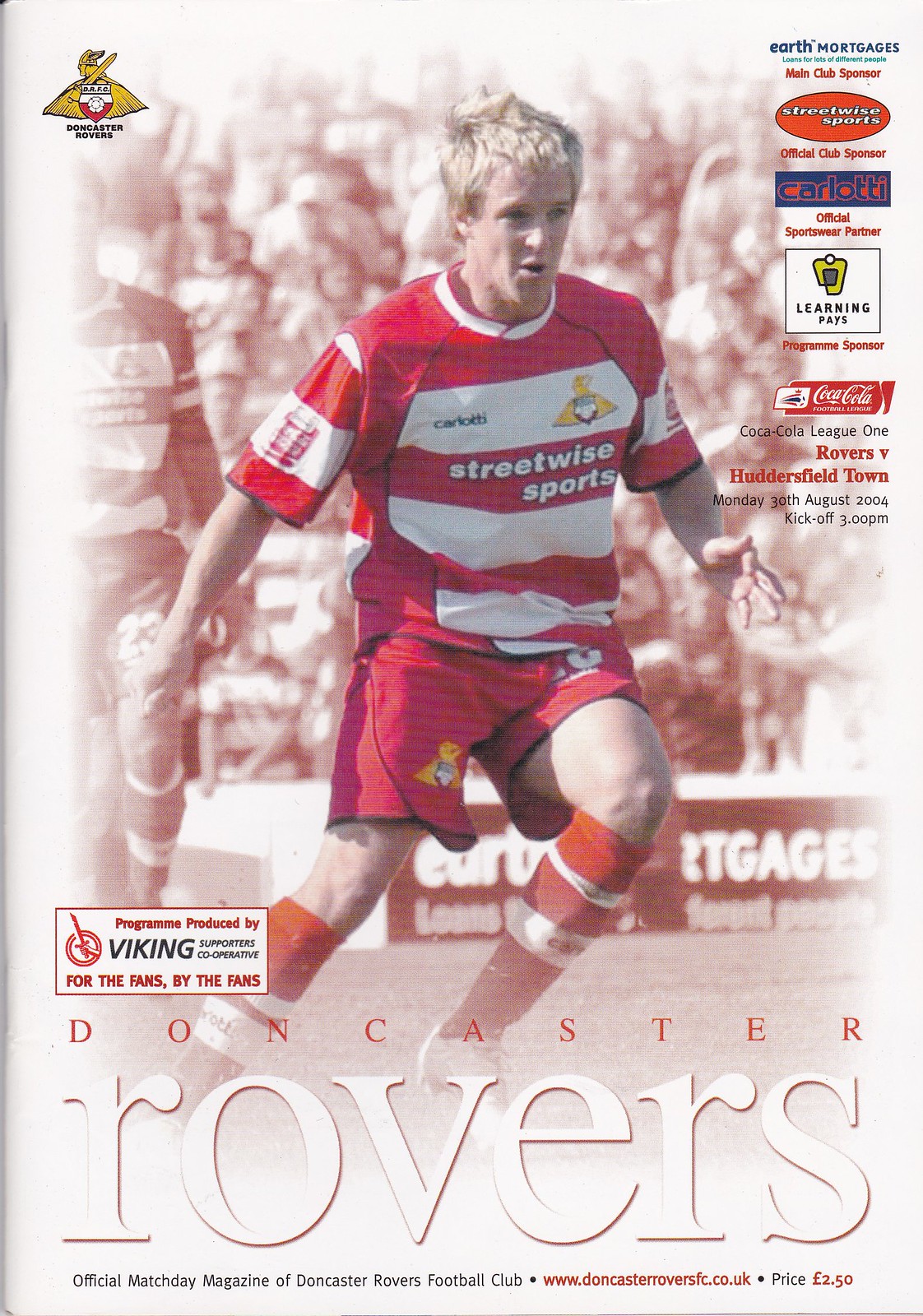The cover of the sports magazine prominently features a vibrant action shot of a soccer player in the center. He wears a red and white striped jersey, red shorts with white accents, and red and white socks. Behind him, another player is barely visible on the left, immersed in the faded and blurry crowd of spectators. The background gradually transitions to a washed-out white, creating a sense of depth.

The focal point player stands out in regular color, contrasting sharply against the predominantly red and white aesthetic. At the bottom of the cover, "Doncaster" is printed in bold red letters, followed by "Rovers" in even larger white letters with a thin red trim beneath it. Additional information includes "Official Matchday Magazine of Doncaster Rovers Football Club" and a website URL, www.doncasterroversfc.co.uk, with a price listed as €2.50.

On the top right corner, logos of various sponsors, such as Coca-Cola and what seems to be an educational foundation named Learning Pays, are stacked vertically. There's also mention of the Coca-Cola League One game: "Rovers vs. Huddersfield Town, Monday 30th August 2004, Kick-off 3.00pm." The overall color scheme, including the background, leans towards light pink, contributing to the magazine's striking visual appeal.